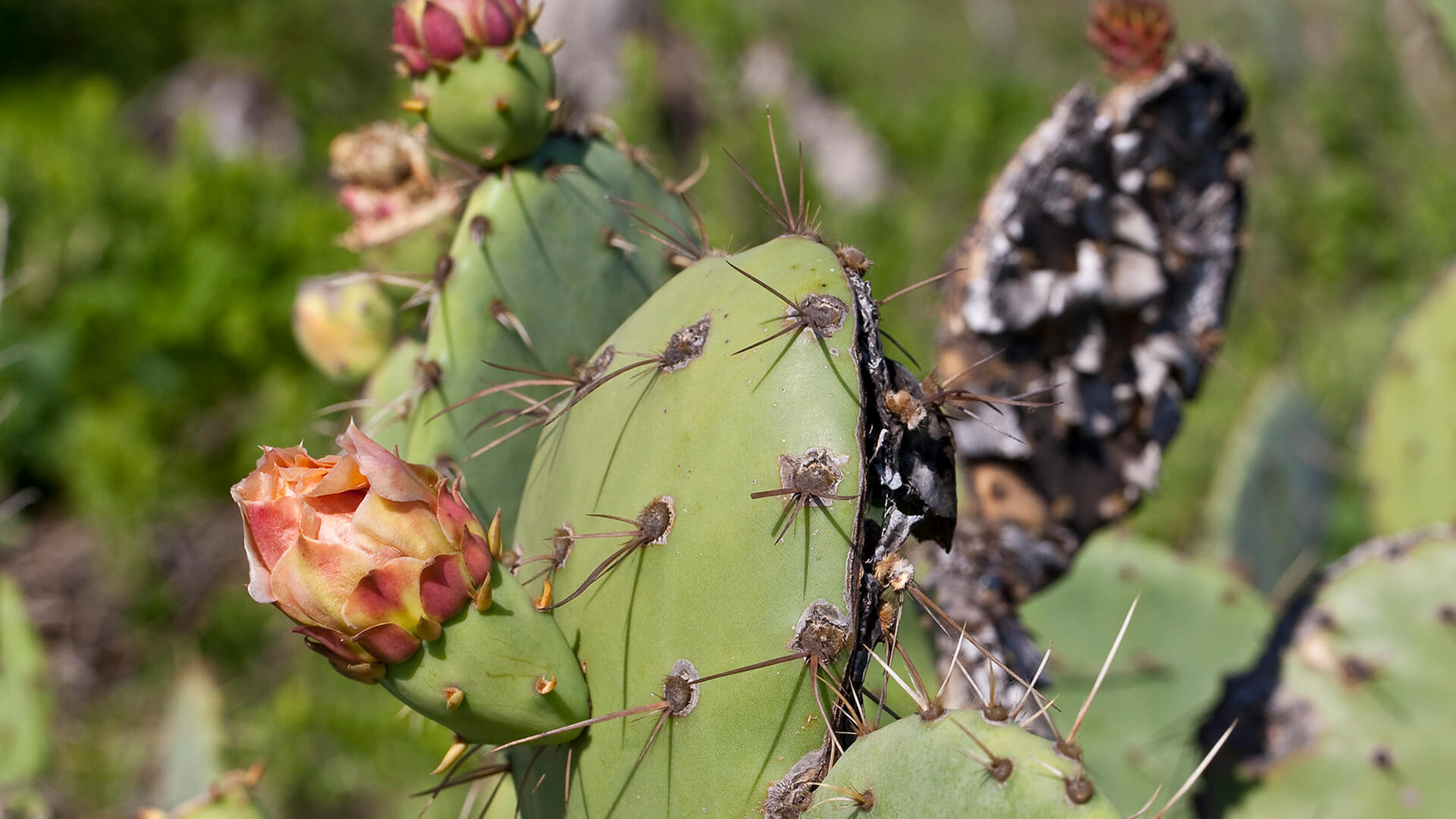In this detailed outdoor photo, the central focus is a striking cactus with flat, round branches. The cactus exhibits an array of vivid blooms, from a light pink with shades of darker pink and yellow on one part, to a striking fuchsia flower on another. The left side of the cactus shows a smaller segment branching out, adorned with closed, pinkish-red flower buds and soft, yellow spikes. Surrounding this segment are darker, longer spines of a brownish-gray hue. Towards the top left, you see another branch with flowers sprouting along its edge, while the furthermost right section of the cactus appears blackened, indicating decay with a reddish-brown or burnt flower. In the center of the cactus is a conspicuous bulb that sports shades of red and yellow. An insect, black and gray, is perched on one of the cactus sections. The backdrop of the image is blurred, dominated by a green hue, with the outlines of other cacti faintly visible, and patches of ground peeking through on the left.